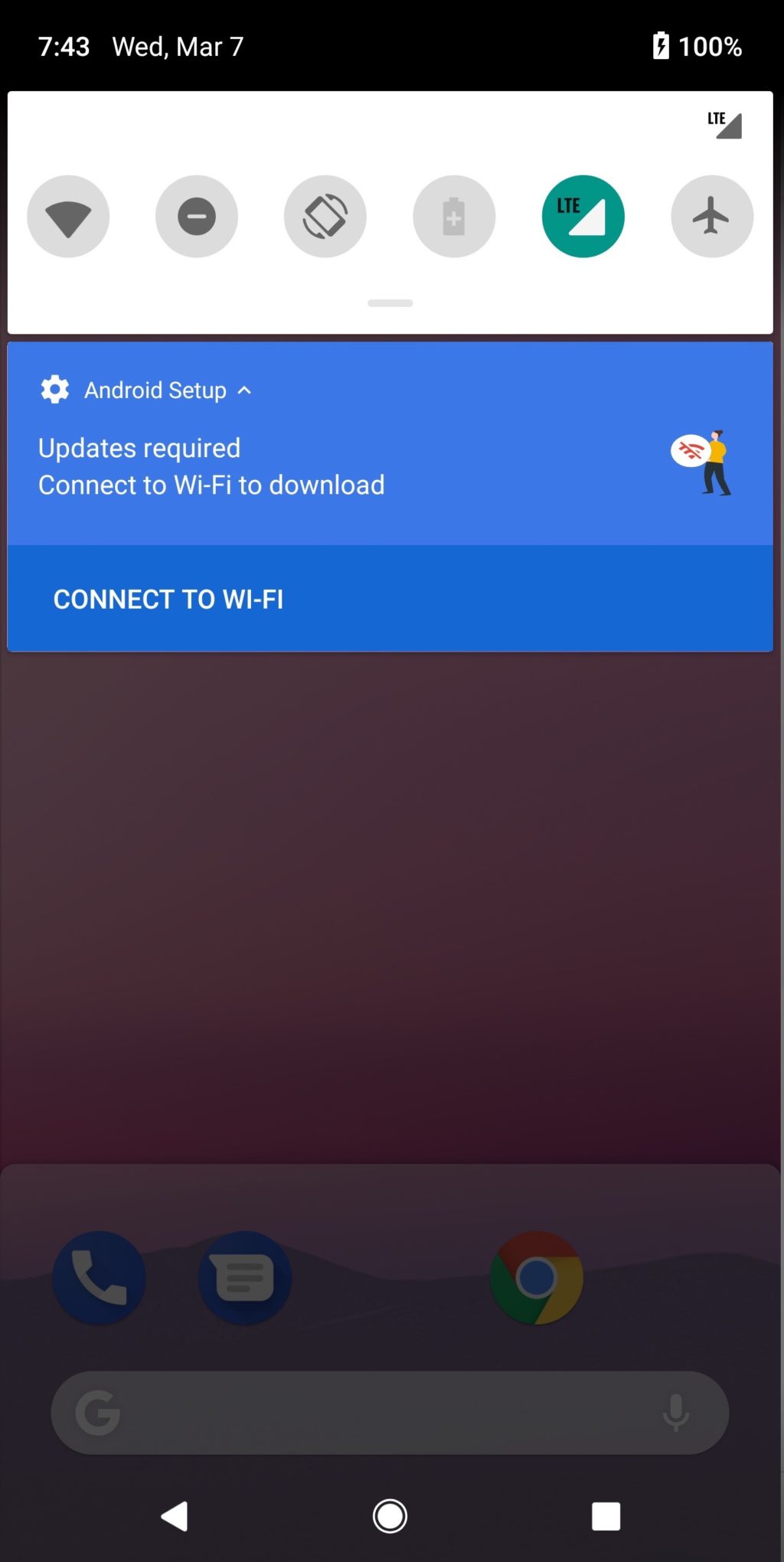In this image, we have a detailed screenshot taken from a mobile device displaying the settings menu pulled down from the top. The quick settings icons visible include Wi-Fi, a minus symbol, auto-rotate, battery saver, cellular signal, LTE, and airplane mode. The time is shown in the upper left corner at 7:43, with the date below as Wednesday, March 7th. The battery indicator in the upper right corner shows a full charge at 100% and currently charging. 

Beneath the top menu, a blue bar labeled "Android setup" reads "Updates required. Connect to Wi-Fi to download," accompanied by an image of a person holding a Wi-Fi symbol with a cross through it, indicating the absence of a Wi-Fi connection. Below, another blue bar urges the user to "Connect to Wi-Fi" in white text. At the bottom of the screen, the phone's home screen is partially visible, showcasing the icons for Phone, Messaging, and Google Chrome.